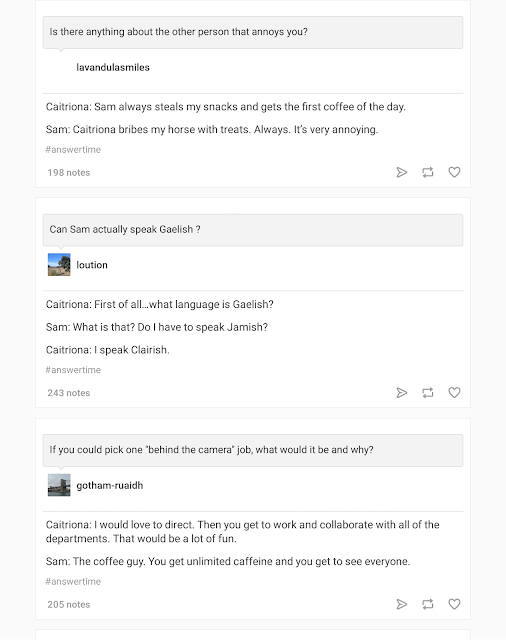This image is a detailed screenshot of an online question-and-answer forum, likely sourced from a social media platform or a comment section under an article. The webpage is designed with a light gray navigation bar at the top, and the text is displayed in black font.

At the forefront, a user named Imdelsmiles has posted a question that reads: “Is there anything about the other person that annoys you?” In response, another user amusingly complains about someone named Sam, detailing how Sam habitually steals their snacks, always gets the first coffee of the day, and bribes their horse with treats, which they find very annoying. This comment has gathered significant interaction with 192 votes.

Following this, a humorous and somewhat perplexing exchange unfolds regarding whether Sam can speak "Gaelish." A user inquires about this language, receiving a playful and cryptic response involving mentions of “Jamish” and “Clarish,” suggesting these might be insider jokes among the participants. This comment thread has garnered 243 likes, indicating it is quite popular among viewers.

Additionally, another question on the forum asks, “If you can pick one behind-the-camera job, what would it be and why?” A user named Gotham replies that they would love to direct, citing the opportunity to work and collaborate with all departments as a compelling reason. Another respondent whimsically suggests that they would prefer the role of the "coffee guy" for the perks of unlimited caffeine and the chance to interact with everyone on set.

The screenshot captures a lively discussion with a white background and black lettering, showcasing various users engaging in a blend of serious and humorous exchanges.